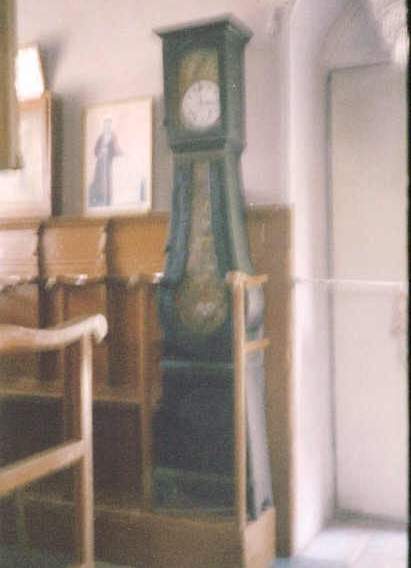The image shows a closed white door on the right side. To the left of the door, there are pew-like wooden seats commonly seen in churches. These seats are connected together and appear to be very thin. In front of these seats, there is a distinctive grandfather clock made of very dark wood. This clock has an unusual design, featuring a single pendulum visible at the front, a clock face at the top, and actually two clock faces—one white and another antique white behind it. The clock has a wide, angular base that slopes gently, reminiscent of a pyramid. The entire scene, including the clock face, appears blurred. Additionally, there seems to be another similar set of seats facing the grandfather clock on the opposite side, creating a sort of symmetrical arrangement.